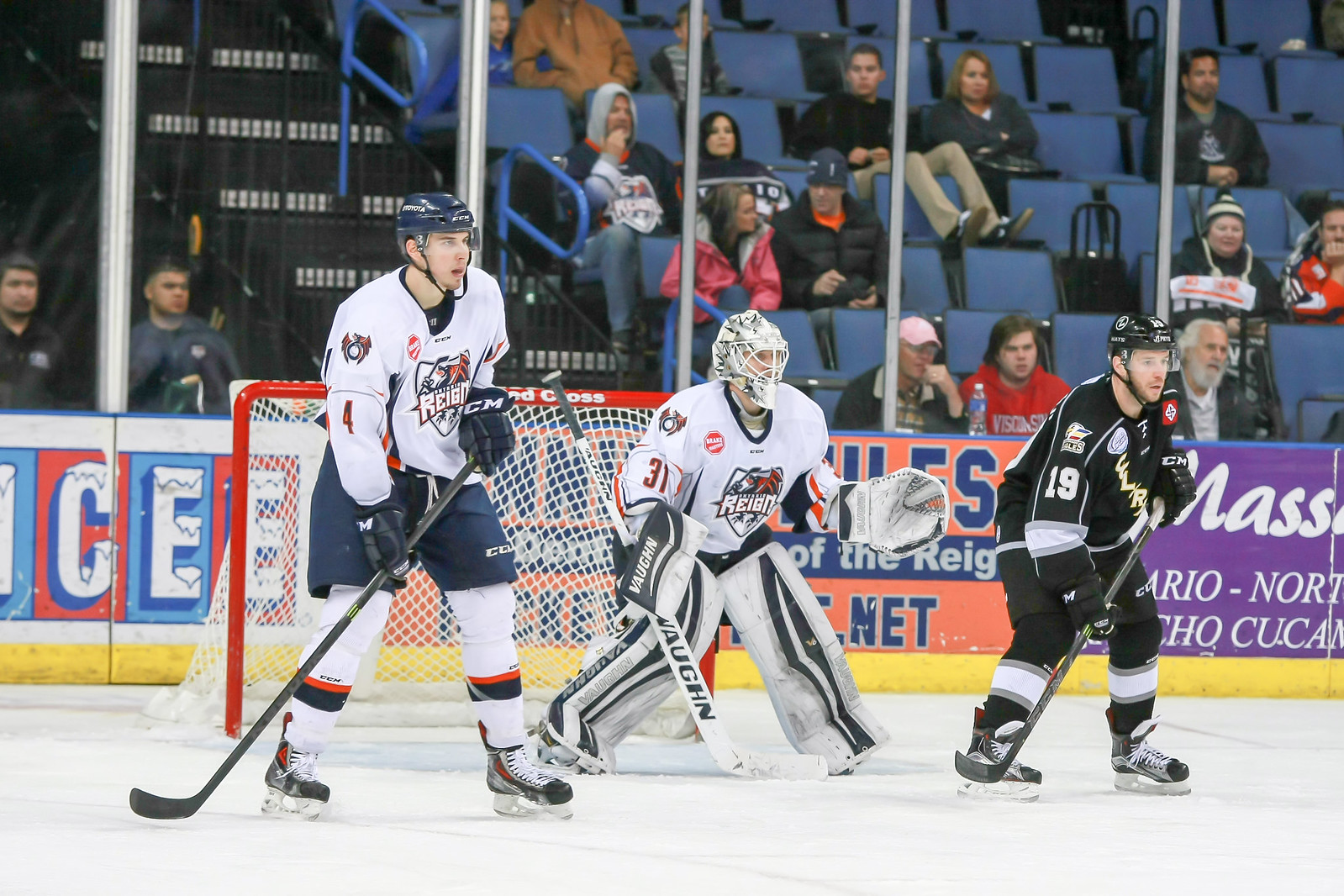The photograph captures three hockey players standing on the ice rink in front of the white net. They are dressed in full hockey gear, with the goalie in the middle donning a predominantly white uniform with protective armor, including a full-face helmet. To his left, another player wears a black uniform, and to his right, a player is dressed in a mix of blue pants and a white top. Each player holds a hockey stick. Behind them, the stadium's wall features various advertisements, including a prominent ICY logo on the left and signs reading "MASS" and another red and blue ad partially obscured by the players. The background shows the rink’s plexiglass barrier and the stadium’s seating area filled with spectators, seated in rows of dark and light blue seats, watching the game intently.